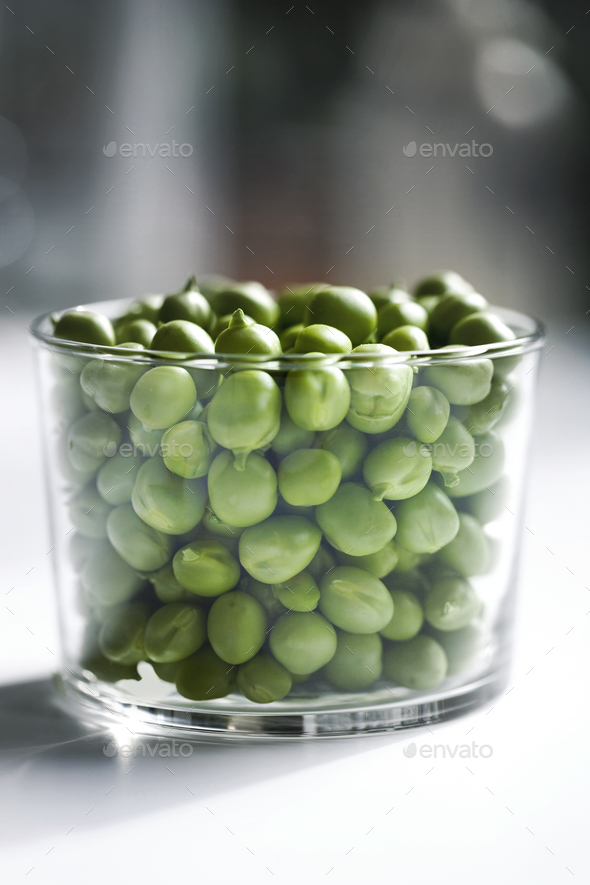This close-up image features a small cylindrical glass bowl filled with shelled green peas, positioned centrally on a white tabletop. The glass bowl appears clear and transparent, offering a detailed view of the vibrant green peas, which are large and spherical, reminiscent of grapes upon first glance. The kitchen-like setting is indicated by the indistinct, gray-blurred background, adding a sense of indoor ambiance. Light, presumably from a right-hand source, casts a distinct shadow diagonally from the bottom right of the bowl towards the back, creating a soft glare at the base of the glass. The presence of the word "Envato," scattered four to six times throughout the image, is subtle but noticeable. The overall color palette is composed of greens, whites, grays, blacks, and browns, contributing to the detailed, yet harmonious depiction of this kitchen scene.